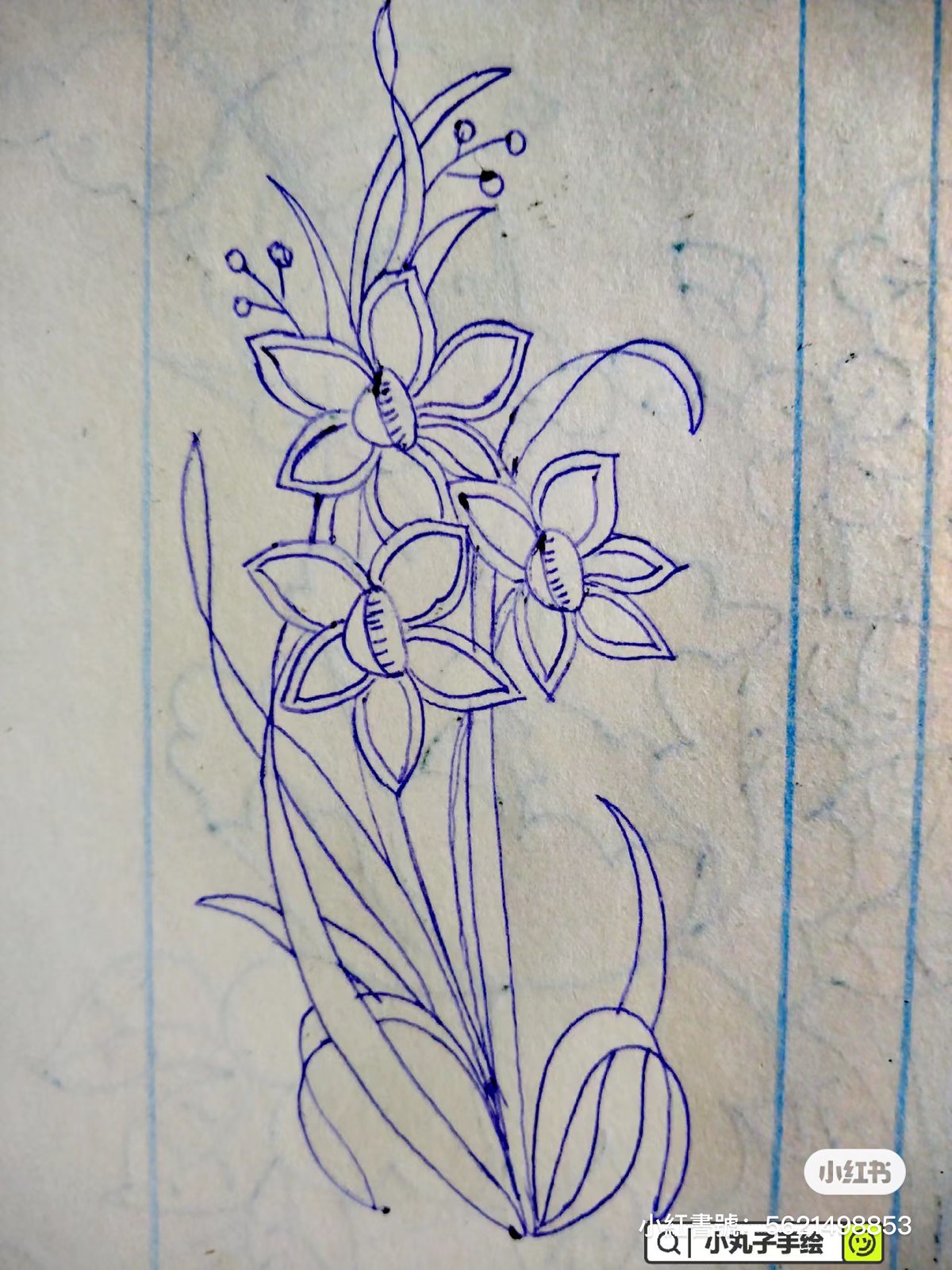The image captures a color photograph of a white piece of paper adorned with intricate blue ink pen drawings. The paper itself features turquoise lines on the right-hand side and a single blue line on the left, resembling notebook paper. In the center of the paper, there's a detailed floral illustration. This drawing has a central stem with thin, slender leaves extending upwards. From the main stem, three smaller stems branch out, each adorned with delicate five-petal flowers. The petals are teardrop-shaped, encircling a circular center with intricate details. Surrounding these primary flowers, small berry-like elements add to the complexity of the artwork. At the bottom right corner of the page is a rectangular block containing black Kanji characters, alongside another green square with an orange edge and a small smiley face. The overall composition suggests a combination of botanical elegance and subtle oriental influences, captured meticulously on what looks to be notebook paper.